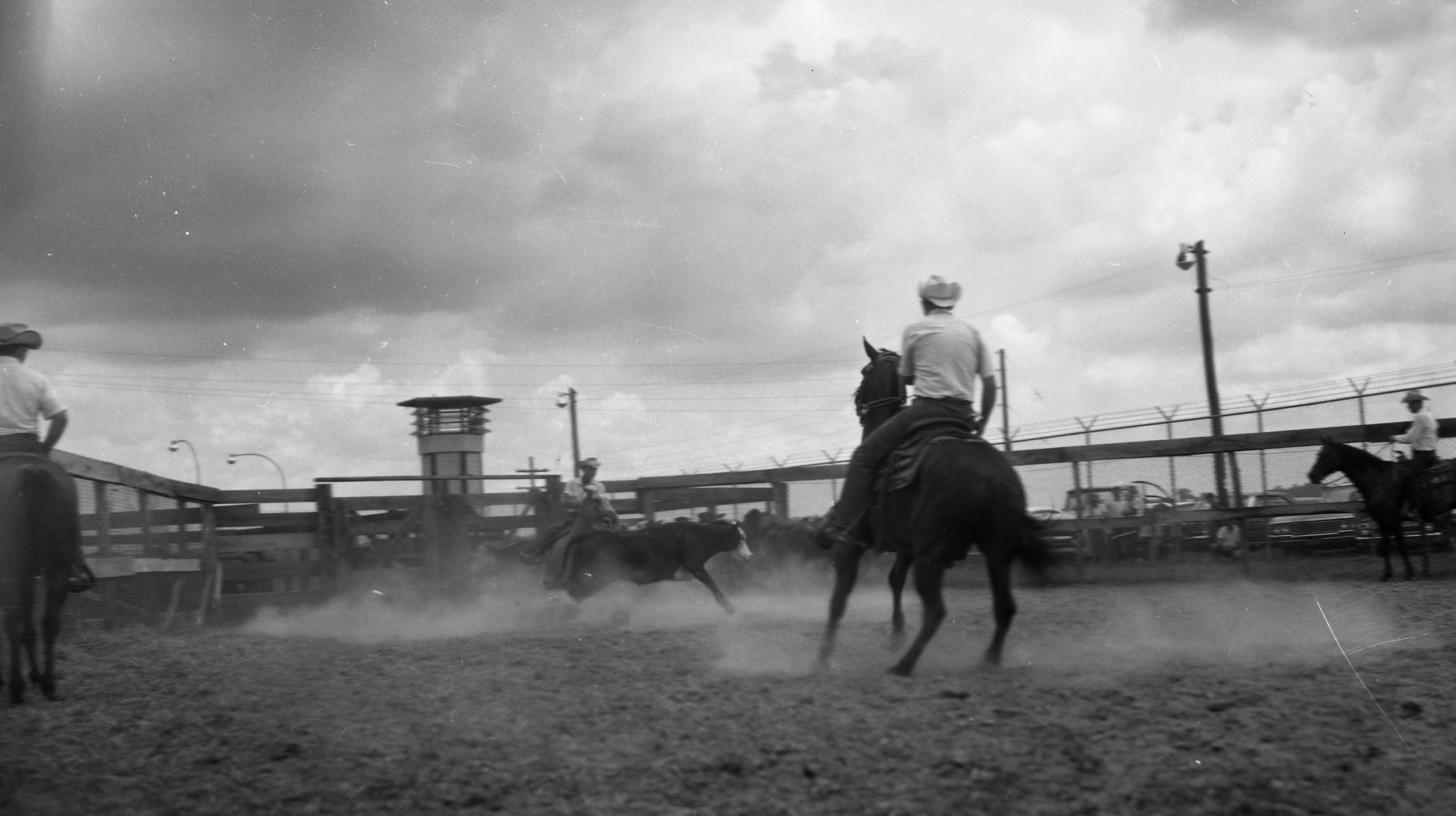In this detailed black and white photo of a lively rodeo in progress, the sky is densely filled with a mix of dark and white billowed clouds, leaving little visible blue. The scene is set within a dirt-filled enclosure, bordered by a combination of wooden and barbed fencing. At the heart of the action, a dust cloud envelops a dark bull being ridden by an unseen rider. Surrounding the bull are four cowboys on horses, all clad in white shirts, black pants, and white cowboy hats. One prominent cowboy on a dark horse, positioned centrally, draws immediate attention. To his left, half-visible, is another cowboy (or possibly a cowgirl), similarly attired. In the background, a stationary cowboy sits on his horse by the right fence, observing the scene. Additionally, behind the rodeo yard, a tower resembling a guard's tower rises above, accompanied by a large, probable light pole. The entire scene conveys the intensity and tradition of rodeo with its dynamic composition and authentic details.